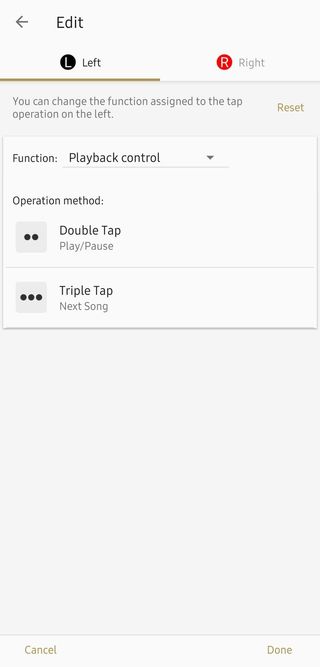The image displays a section of a web interface focused predominantly on the upper half of the screen. In the upper left corner, there is an "Edit" button accompanied by a left-pointing arrow. Adjacent to this, on the left side, is a black circle containing the letter "L" for left, and on the right, a red circle with an "R" for right. The left option is underlined with a brown bar, indicating it is selected. Below this, instructional text reads, "You can change the function assigned to the tap operation on the left." 

In a rusty brown color, there is a "Reset" button followed by another line of text stating "Function: Playback Control" with a dropdown arrow next to it. This section is faintly underlined with light gray.

Further down, there is a segment labeled "Operation Method" accompanied by "Double Tap". To the left of this text, an illustration in a light gray box features two round black dots labeled "Play/Pause". Below this box, a gray horizontal line separates the next operation, "Triple Tap," from which the text "Next Song" appears in light gray. This is accompanied by another light gray box depicting three black dots.

The lower portion of the image is blank, culminating in a bottom row that contains two buttons labeled "Cancel" and "Done," each presented in a brown color.